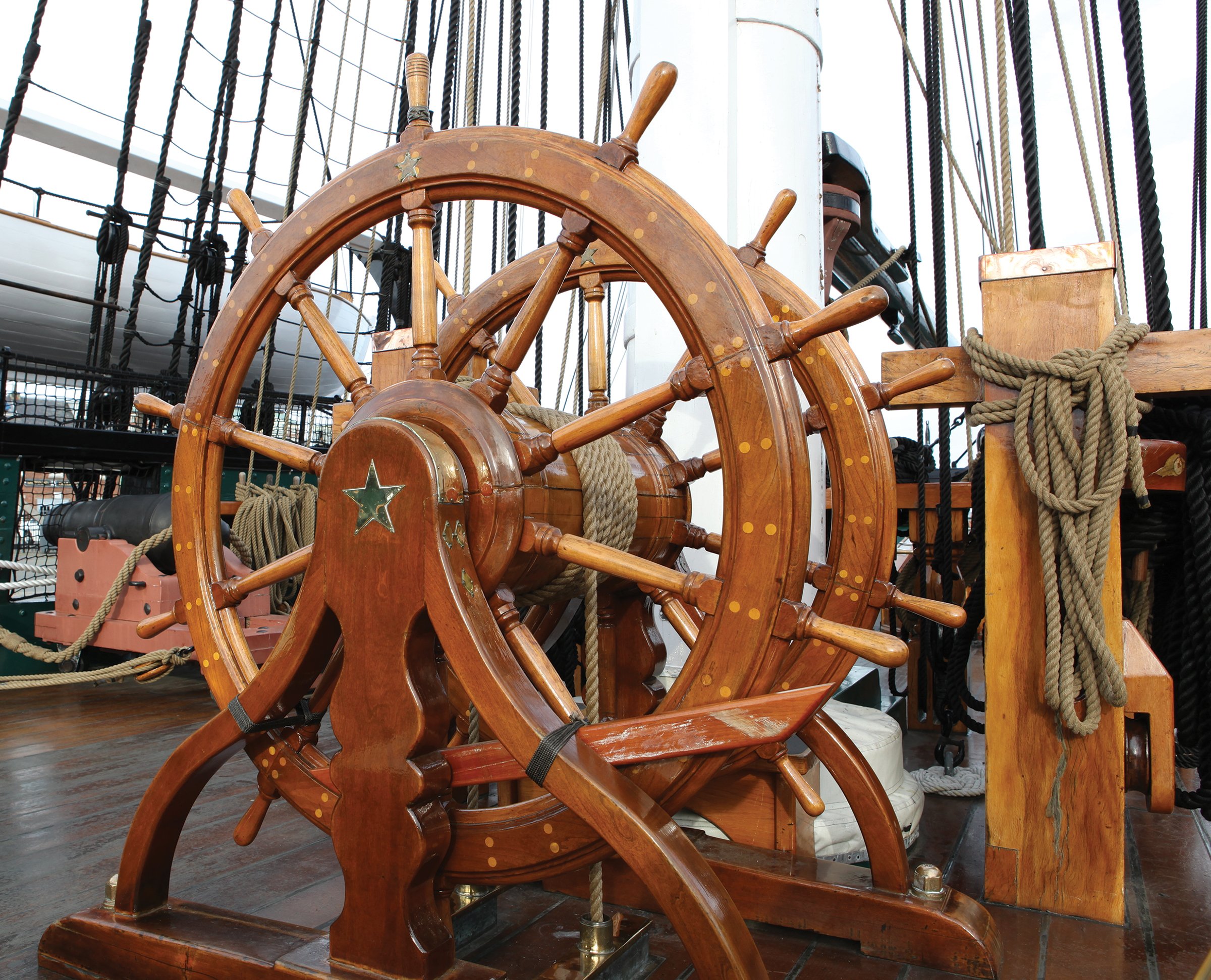The image depicts the deck of an old wooden sailing ship, centered around a large, double wooden steering wheel adorned with a gold star on its frame. Both wheels, connected by a cylindrical wooden tube wrapped in rope, feature multiple spokes and handles. The deck is made of dark, stained wood that looks well-maintained, contrasted by the lighter tone of the wheels. To the right of the wheels, a post and beam structure supports ropes and rigging, typical for sail manipulation. In the background, white tubing, which might be plastic or painted metal, extends out of the frame, possibly part of the ship's crane or other equipment. A notable feature to the side is a mounted cannon on a wooden platform, with thick rope draped over it. The sky above is overcast, enhancing the historic and aged aesthetic of the ship. Overall, the intricate details of the wheels, deck, and rigging evoke the ship's purpose and era.